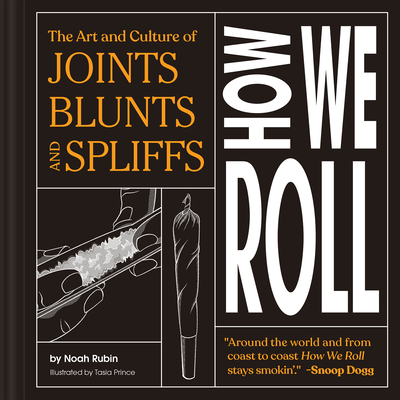This image depicts a book cover with a square, predominantly black background. The right edge of the cover features a subtle indent, mimicking the spine of a book. Centered, but slightly offset to the right, is a thin white outline of a square, within which the book's decoration is sectioned into smaller rectangles. The upper left corner of the cover boasts the title "The Art and Culture of Joints, Blunts, and Spliffs" in bold orange letters. Below this title, there are detailed illustrations in white of a joint and a hand rolling a blunt. Towards the bottom left, the book credits "By Noah Rubin, Illustrated by Tasia Prince" are visible. The right side of the cover prominently displays the phrase "How We Roll" in large white letters. At the lower right corner, an orange quote reads, "Around the world and from coast to coast, how we roll. Stay smokin'." followed by Snoop Dogg's endorsement. The overall design, coupled with the thematic illustrations and quotes, suggests a comprehensive guide or cultural exploration of marijuana rolling practices.